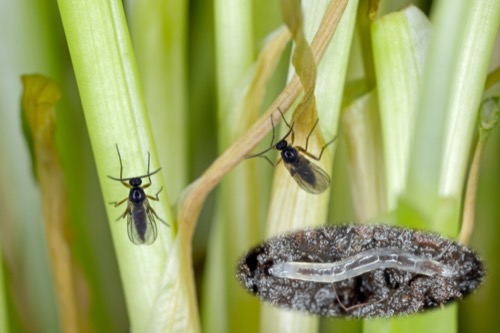In this detailed close-up photograph, two black ants are climbing up the yellowish-green stalks of a plant that resembles bamboo, though some have compared it to the layered structure of green onions. The plant consists of multiple stalks, which blur into the background, emphasizing the clear focus on the ants. The image is taken from a front point of view, highlighting the ants as they traverse the stalks. In the bottom right-hand corner, there's a zoomed-in cutaway showing a bacteria inside a black cell, positioned on two of the stalks. This bacteria is presented in striking contrast to the rest of the image and adds an unexpected element. The ants' movement and the bacteria's presence suggest an intricate relationship, although the exact context remains undefined due to the absence of additional information. The depth of field makes the background stalks appear blurry, ensuring the primary focus stays on the detailed subjects in the foreground.